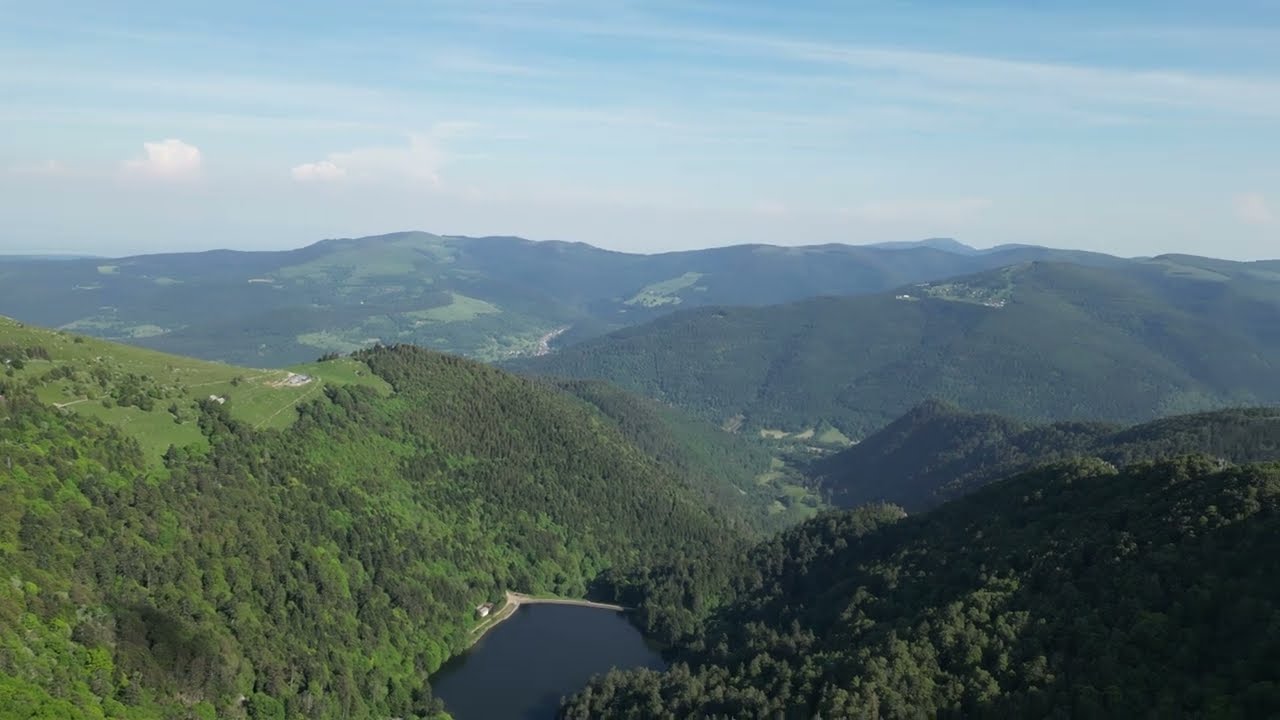This aerial photograph captures a lush, hilly landscape dominated by verdant, tree-covered hills and interspersed with patches of short grass and pastures. At the bottom of the image lies a small pond or lake with dark, deep blue water, bordered by sporadic hints of man-made structures, including a possible house or building near the water's edge and maybe some buildings atop a hill on the left. The sky above is predominantly blue, graced with wispy cirrus clouds and sporadic puffy white clouds, contributing to the mostly sunny atmosphere. In some areas, the green gives way to brown strips, potentially indicating roads. The scenery is striking in its greenery, lacking the rocky or snowy characteristics often associated with mountainous regions, and overall, it renders a picturesque and serene natural vista.